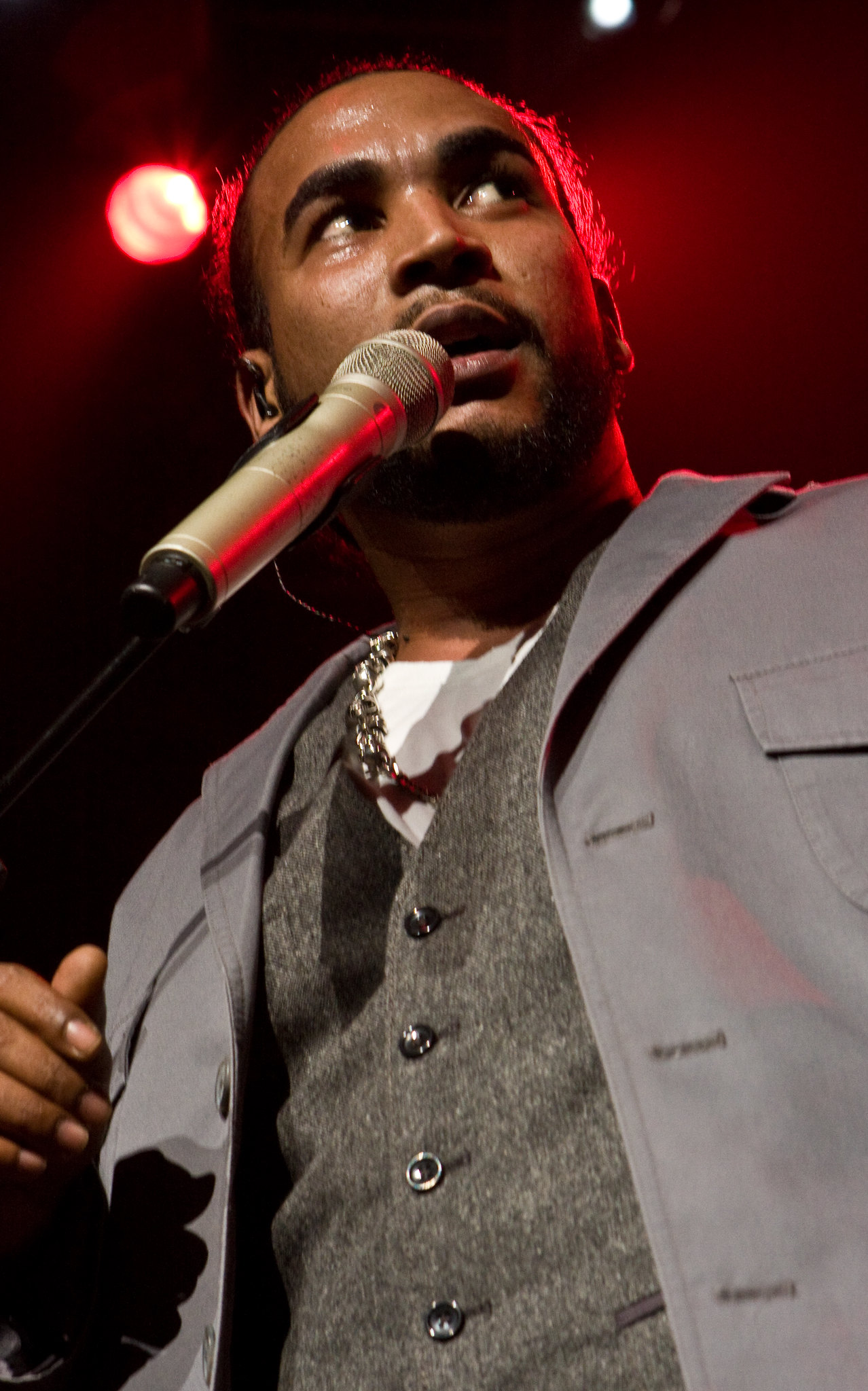The professionally taken photo captures an upward angle of an African-American or Latino man in mid-performance, either singing or speaking into a microphone. He's on a stage illuminated by overhead spotlights that cast shades of red and pink. The man, whose hair is tied up and who has some facial hair, is dressed in a light blue jacket over a gray button-down vest and a white shirt, with a chunky silver chain around his neck. He appears slightly sweaty, emphasizing the intensity of his performance. He is looking off to the right, with an ear monitor in his visible right ear, and his left hand is raised as though holding the microphone, though the stand isn't visible. The scene suggests a concert or performance setting, with the focus solely on the performer against a vibrant backdrop of varied colors, including black, white, gray, light blue, red, and pink.